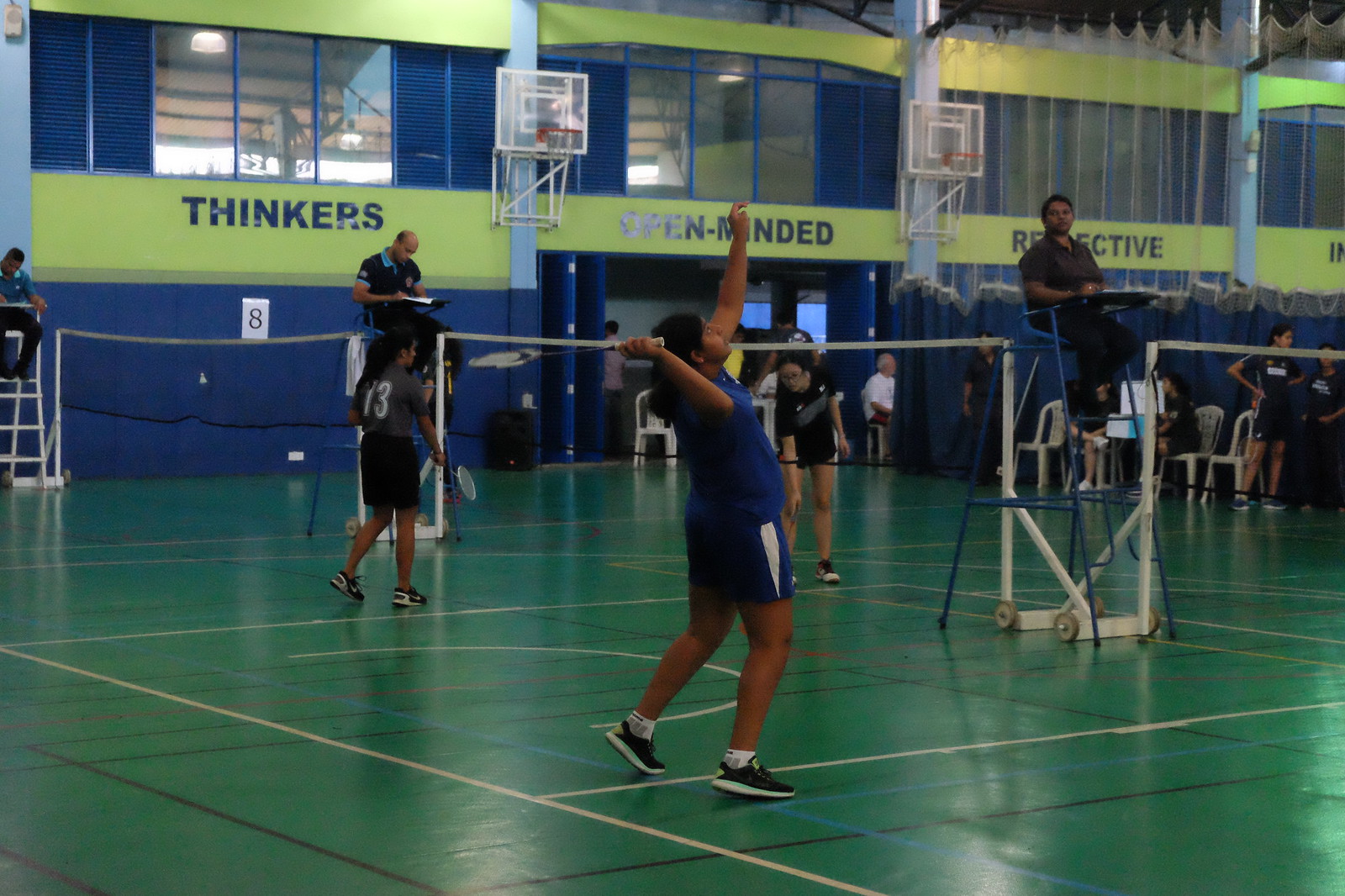This full-color indoor photograph captures a vibrant badminton tournament set in a high school gymnasium. Several young female players, distinguished by their longer hair, are actively engaged in matches across three courts with white badminton nets. The gym features a green floor adorned with white, blue, and black lines, and is edged with blue walls accented by lime-yellow or fluorescent yellow stripes. Basketball nets are folded up against the walls, reinforcing the multipurpose use of the space. Elevated chairs hold referees clad in varied uniforms—one in a gray shirt and black pants on a blue chair with a white frame, another in a blue shirt, and a third in a black shirt with blue lapels. The gym walls are decorated with the words "Thinkers" and "Open-minded Perspective" in blue letters against a yellow band. Illuminated by daylight streaming through the windows, the scene is dynamic and lively, with an audience in white chairs and blue curtains surrounding the courts. The nearest player, poised to serve the birdie, wears a blue uniform with white stripes on her shorts and black and white shoes. Other players visible include one in a gray shirt and black shorts with the number 13 in white, and another in black and white with glasses, adding to the spirited atmosphere of the event.